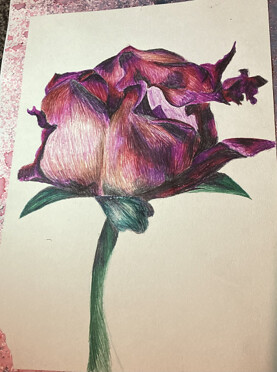This is a photograph featuring a hand-drawn illustration of a flower, resembling a rose, rendered in a vibrant, colorful style. The flower, showcased on a beige sheet of paper, displays various shades of pink, purple, and deep red, with parts of the petals and stem appearing unfinished or less defined. A notable detail is the top right petal, which has a face-like appearance and seems to be tearing or flayed. The green stem exhibits a mossy tint, with some areas not fully shaded, revealing a gray outline. The background consists of a white and burgundy mosaic or speckled pattern that likely belongs to a table, introducing some shadows across the sheet of paper. There is no signature on the drawing, enhancing the focus on the intricate and expressive depiction of the flower.